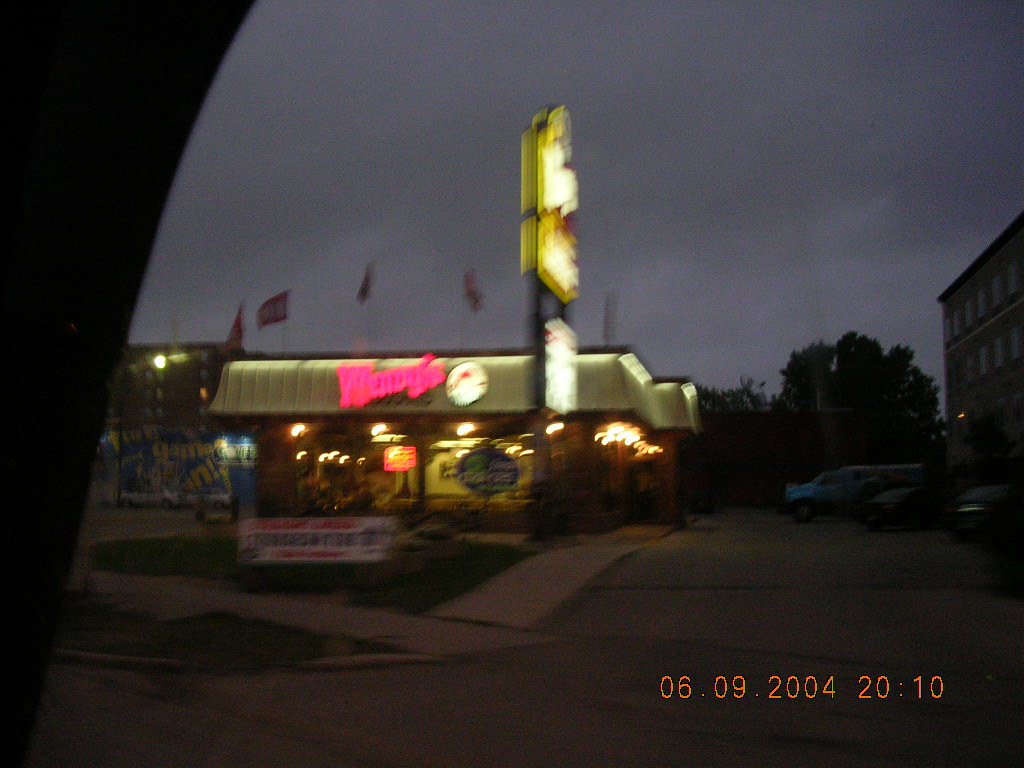The photograph, taken in the evening or near nighttime, depicts a bustling, yet grainy outdoor scene dominated by a Wendy's restaurant. The dark and cloudy sky hints at the late hour, while the bright, illuminated signage of Wendy's stands out against the gloomy backdrop. The image is blurred and grainy, suggesting it might have been taken from inside a car, evident from the partial view of what appears to be the curved edge of a window on the left.

In the foreground, a small portion of lawn features an illegible white sign with black and red text due to the blur. The restaurant's lights are vivid and the interior appears open, showcasing a beige roof and large glass windows adorned with various signs and lights. These lights exhibit a bokeh effect, suggesting motion during the photo capture.

To the right, indistinct parked vehicles, including what looks like a blue truck and several sedans, line the area near the building. The parking lot stretches towards the viewer, adding depth to the scene. On the left side of the Wendy's, an indistinguishable structure looms, shrouded in darkness.

Adorning the roof are five red flags, their details lost to the blur. A prominent Wendy's sign and another large sign in the distinctive logo shape anchor the scene. The bottom right corner of the image features an orange timestamp "06.09.2004 20:10", suggesting the photo was taken on June 9th, 2004 at 8:10 PM.